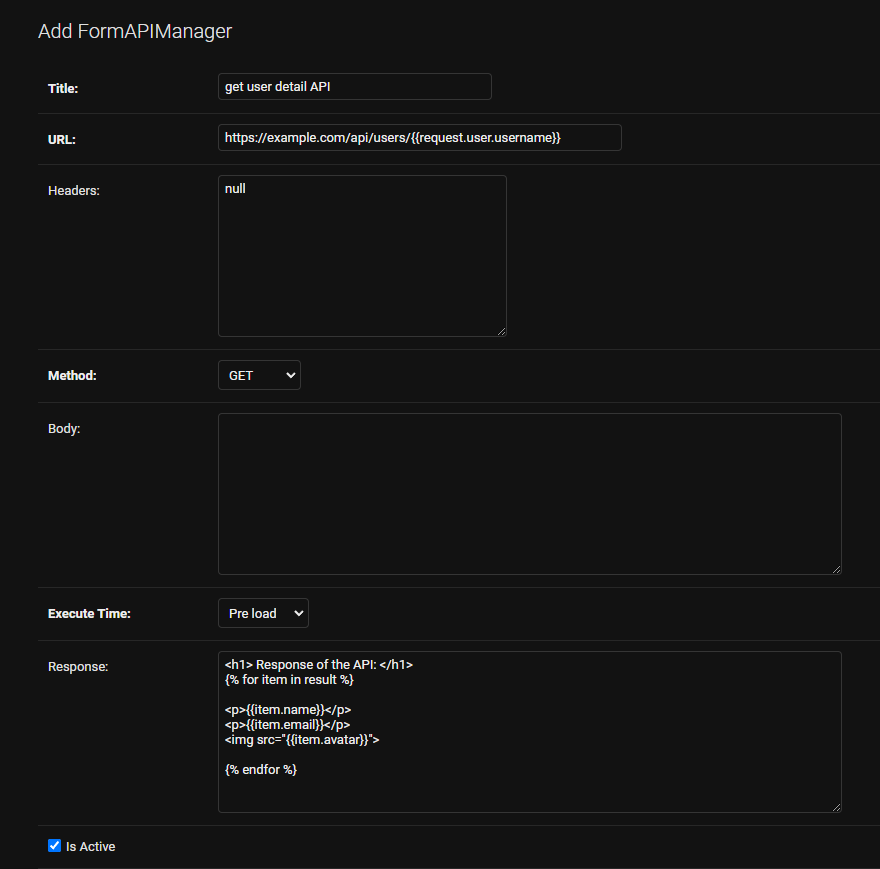The image displays a black-background interface page, prominently featuring a top-left corner title that reads, "Add Form API Manager." The layout includes a structured form with labeled fields to input various types of information. The labels, listed vertically on the left side, are: "Title," "URL," "Headers," "Method," "Body," "Execute Time," and "Response." 

To the right of each label, specific example content or placeholders are provided. The "Title" field contains the text "Get User Detail API." The "URL" field displays a sample URL, "example.com/api/users/request_user_names." The "Headers" field simply states "null," spelled out as "N-U-L-L." The "Body" field is entirely blank, indicating that no content has been inputted.

At the bottom-left corner of the interface, there is a small blue square with a white check mark inside it, signifying that the user is active.